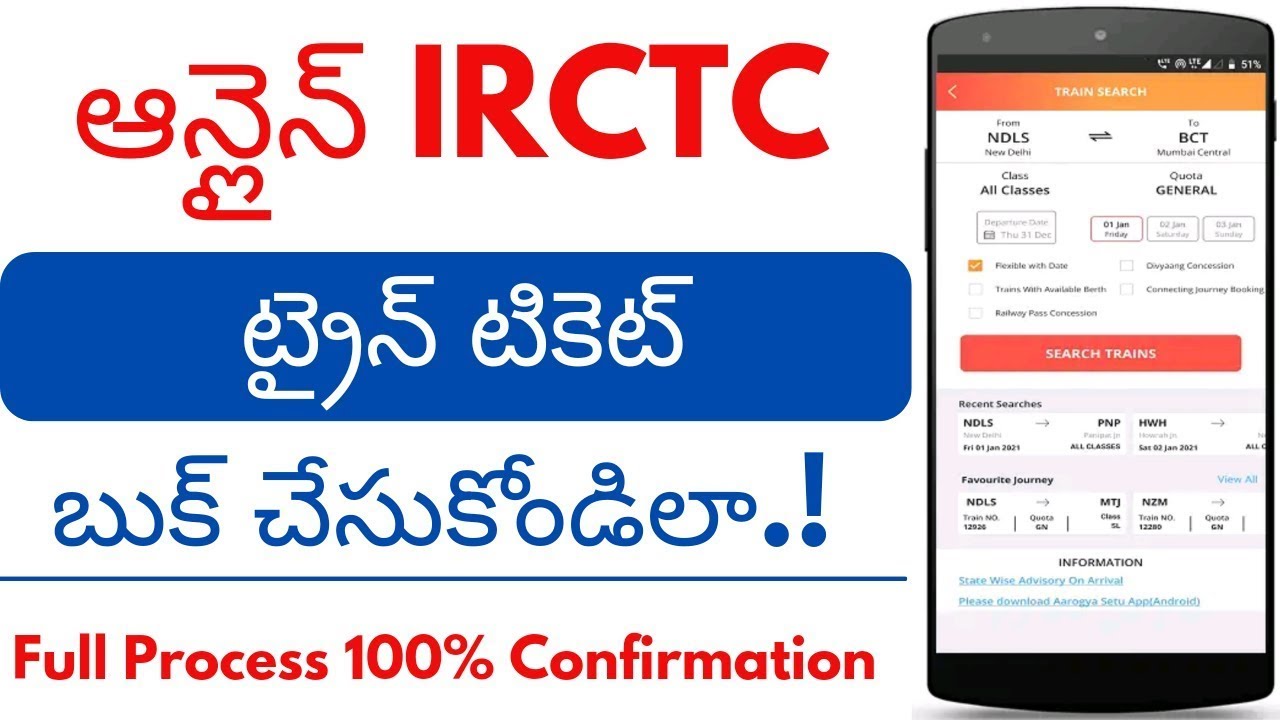This is a screenshot taken from a web browser on a desktop PC showcasing the IRCTC 'Plan My Travel' page. The page is framed by blue borders on the top, left, and right, while the main content area is white. At the very top of the page, the website is identified as "TheTourismTimes.com". In the upper-left corner of the white section, the header reads "Indian Railway Catering and Tourism Corporation Limited" alongside a white and blue emblem. Below this, the page greets the user with "Welcome, Mr. Ravinder Baikon". On the left side, there are labels such as "Opinion Poll" and menu options including "Tour Packages," "Flights," "Hotels," "Tourist Train," "Cabs," and "Loyalty Program." The central part of the page features the "Plan My Travel" section and contains buttons for "Booking History," "Print Ticket," "Cancellation," "Refunds," "Sub Yatra," and "File TDR."